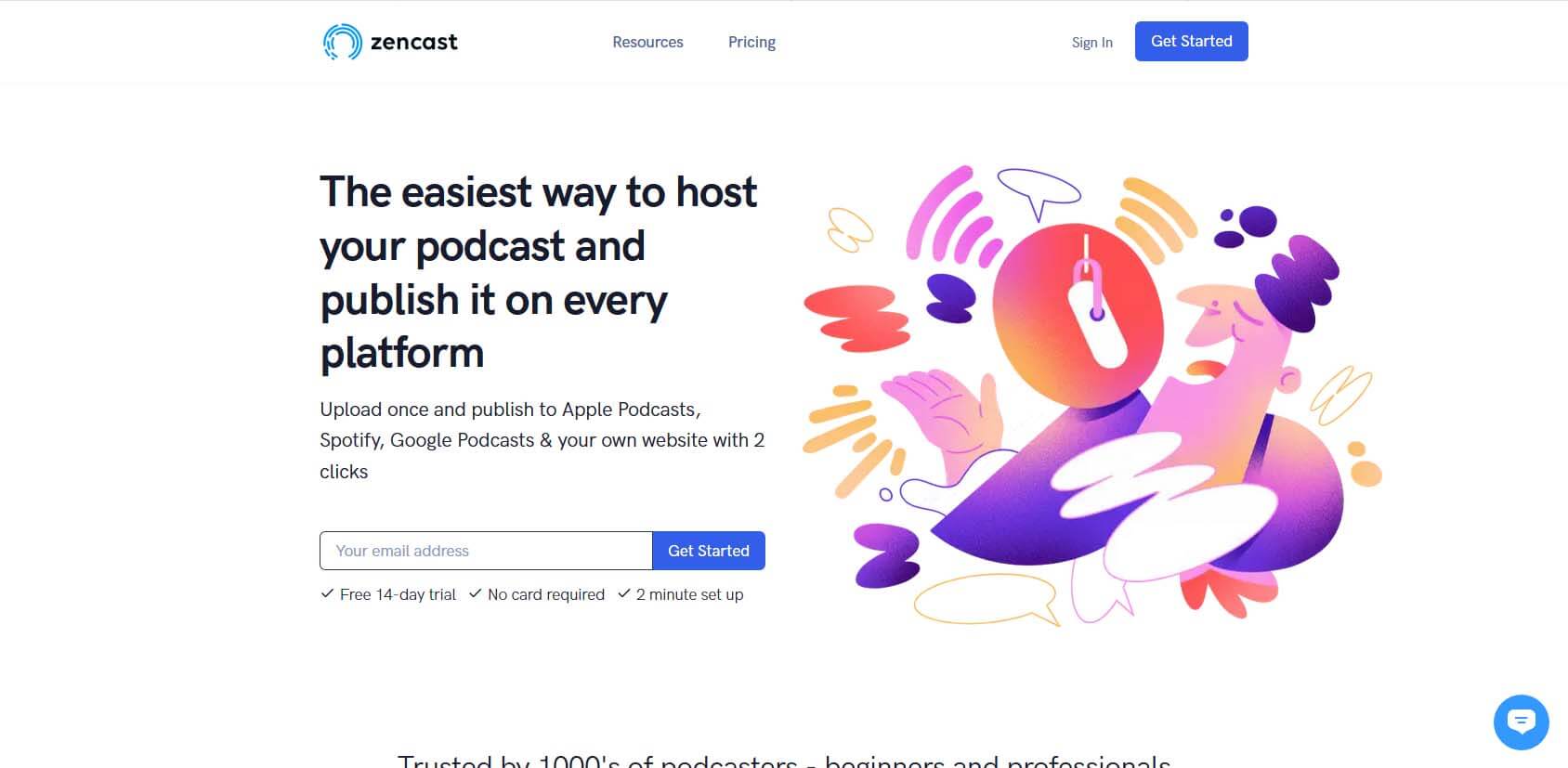This is a detailed screenshot of a web page in portrait orientation, slightly longer than its height. The top of the page features a thin gray horizontal line forming a border, setting off the contents below. At the very top, there is a prominent white box containing a circular blue-and-white logo with the word "Zencast" in black. To the right of the logo are navigation links in gray text, labeled "Resources," "Pricing," and "Sign In." Further to the right is a conspicuous blue rectangular button with white text that reads "Get Started."

Beneath this header, the background predominantly consists of white space. On the left, there is a headline in black text that reads, "The easiest way to host your podcast and publish it on every platform." Below this headline is a gray-text description, followed by a white search box with an adjacent blue button containing the white text "Get Started."

Below this section, a series of bullet points with check marks detail features such as "Free 14-day trial," "No card required," and "2-minute setup." Directly under these features, there is an image depicting a person who appears to be speaking, with their hand extended outward. The background of this image is decorated with numerous text bubbles and WiFi-like signal icons.

Toward the bottom, a partially visible description reads, "Trusted by thousands of podcasters, beginners, and professionals," though the text is cut off. To the right of this description is a small chat icon.

In summary, this screenshot is of a clean, user-friendly web page, designed to attract and guide users interested in hosting and publishing podcasts effortlessly.